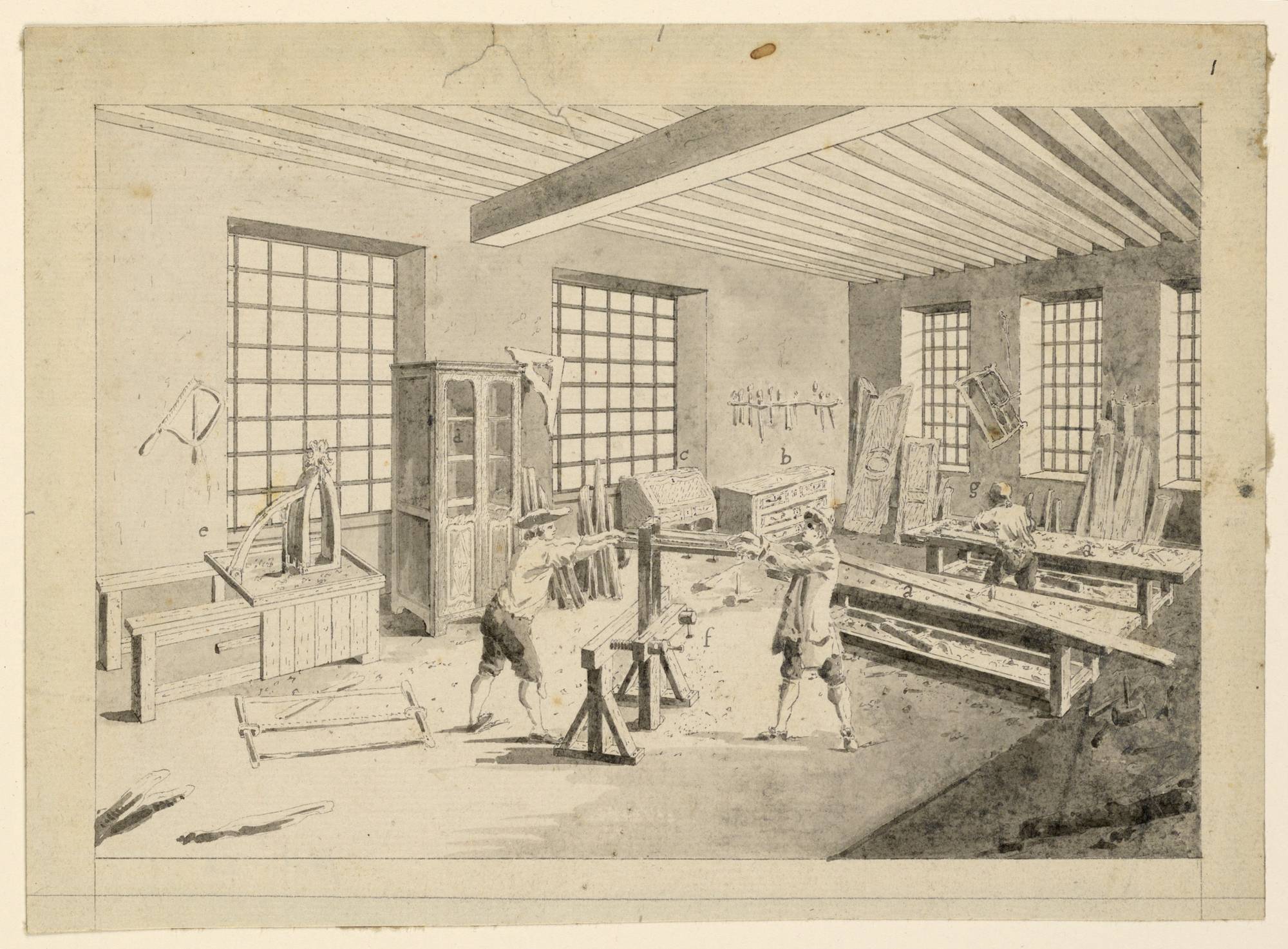This grayscale image, likely an old pencil or line drawing, portrays a detailed carpentry workshop scene that seems aged, with yellowed, frayed edges. Set inside a partially completed or abandoned building with a high wood-beamed ceiling, three men are meticulously engaged in their tasks. Two of them, dressed in historic attire — one in revolutionary garb and the other in knickers and a longer coat — are maneuvering a carpentry machine, possibly a saw, appearing to cut or approach wood. The third man, seated at a table laden with numerous parts, works intently away from the viewer. Surrounding them are various carpentry tools hanging on the walls and scattered on the floor, a large and empty china cabinet, and slanted pictures. Shutters are conspicuously displaced, contributing to the sense of disarray. This image illustrates a working environment steeped in history, possibly during a tumultuous period, encapsulating a vivid moment of productive labor within an architectural workshop.